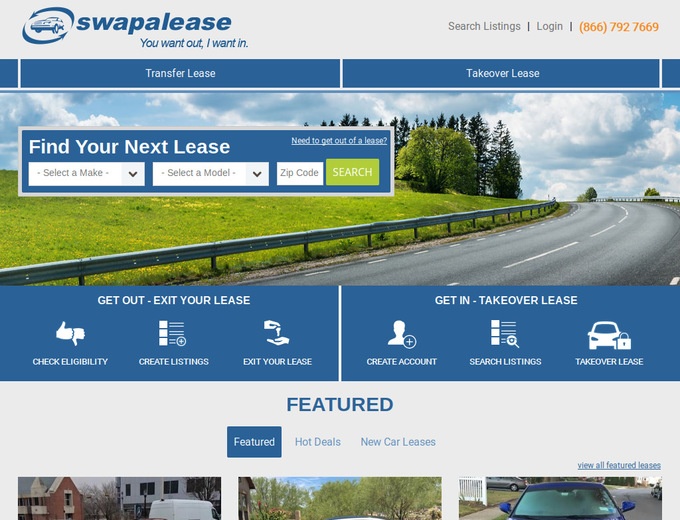This image captures the interface of a website named Swapalease, which specializes in car lease transfers. The main visual focuses on a blue-themed graphic featuring a car encircled by revolving arrows, illustrating the concept of switching or transferring leases. Prominent text on the graphic reads "You want out, I want in," along with directives "Transfer Lease" and "Take Over Lease," though some sections are slightly cropped at the top.

At the top of the screen, the website displays standard navigation options such as "Search Listings" and "Login," along with a phone number highlighted in orange for easy visibility.

Running down the left side of the image, there is a picturesque road curving to the left, lined with lush green grass and framed by an array of trees. The serene backdrop includes a partly cloudy sky with fluffy white clouds against a blue horizon.

Centered within the blue section of the image, the text "Get Out - Exit Your Lease" and "Get In - Take Over Lease" are prominently displayed. Below these headers, additional options are listed: "Check Eligibility," "Create Listings," "Exit Your Lease" on one side, and "Create Account," "Search Listings," "Take Over Lease" on the other.

This detailed snapshot encapsulates the core functionality and services offered by the Swapalease website, enhancing the user's understanding of how they can either transfer out of their current lease or take over someone else's.